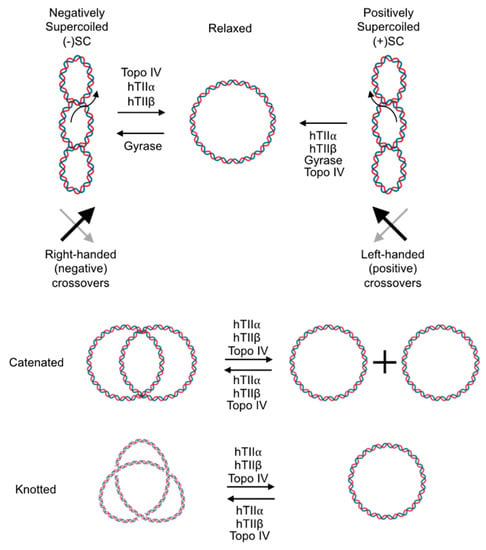The image is a detailed scientific chart, presented in portrait mode with no background, featuring a complex diagram of various intertwined circular and oval shapes. These shapes, composed of wavy, interconnected red and teal-green strands, resemble a double helix pattern. The diagram is segmented and annotated with numerous labels and arrows.

The top left corner reads "negatively supercoiled (SC)," accompanied by three such hoops. Adjacent to this, specific annotations like "topo IV," "HTLLA," "HTLLB," and "GYRASE" are present, with black arrows pointing towards corresponding areas. At the chart's center top, the term "relaxed" is prominently displayed above a large red-green hoop, with several arrows targeting this structure from various labels.

The top right corner mentions "positively supercoiled (+SC)" with three associated hoops beneath it, accompanied by an upward arrow. The bottom left corner describes "knotted," illustrating three interlocked hoops forming a knot. Finally, the bottom right corner shows a single large hoop described as "catenated."

Through this intricate visual representation, the diagram explains various states of supercoiling, crossover orientations, and conformational states like knotted and catenated, using scientific terminologies and clear directional arrows for guidance.